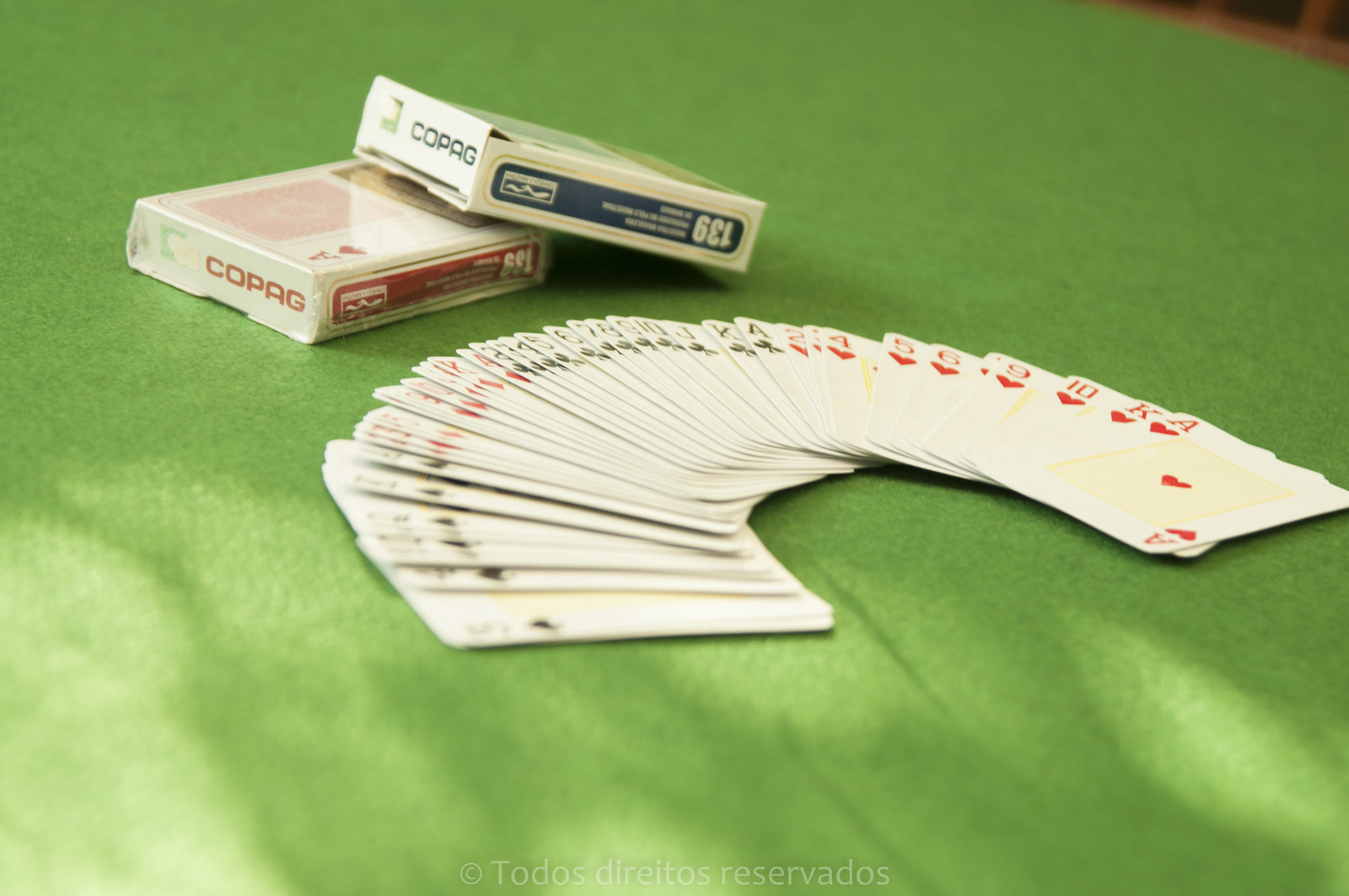The image features a neatly fanned-out deck of playing cards spread across a green table. Positioned slightly on top of each other and to the side of the deck are two boxes that appear to be the packaging for the cards. The top box has blue details and rests partially over the bottom box, which has red details. Both boxes prominently display the brand name "COPENK" and the number "139" on their sides, presumably indicating the quantity of cards each box contains. The text on the red-detailed box is in red, while the text on the blue-detailed box is in blue, consistent with their respective color themes. The scene suggests a gathering where people are engaged in playing cards.